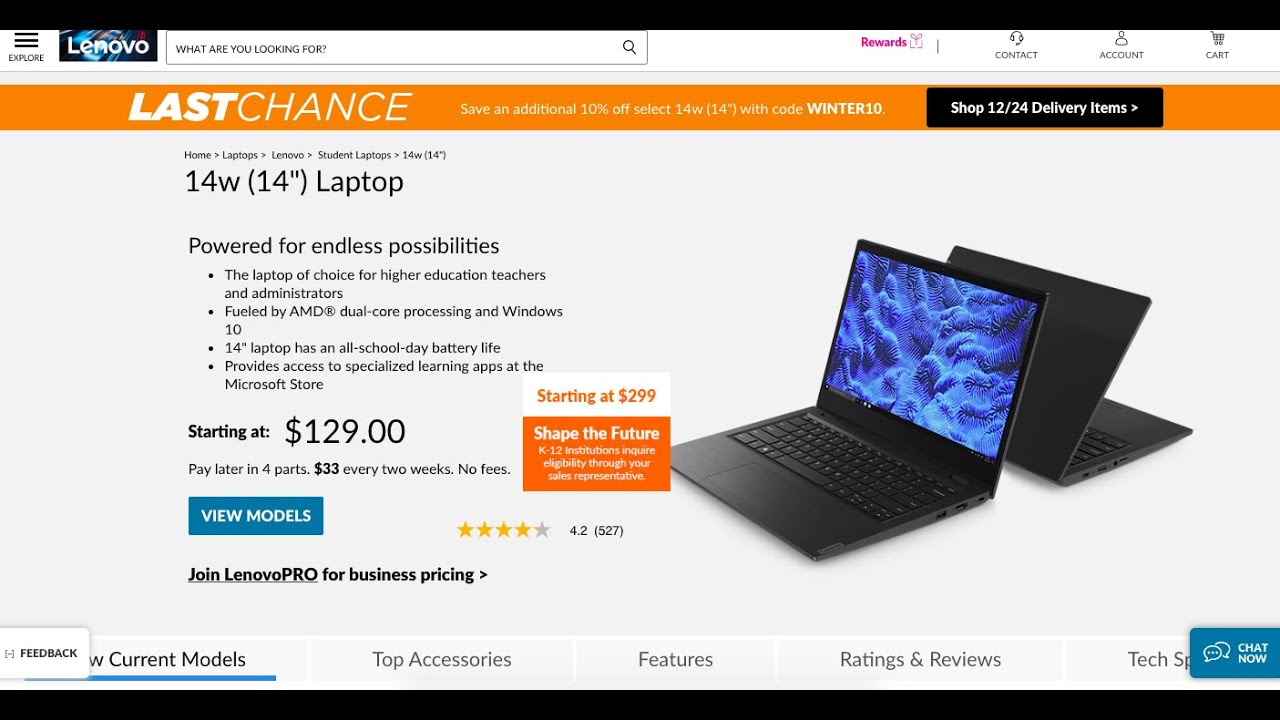The image is a screenshot of the "Last Chance" webpage from the Lenovo website. 

The layout begins with a black background band running across the top of the page. On the top left is a navigation button, and to its right is a Lenovo advertisement. Further along to the right, there is a search bar, next to which is a pink text link labeled "Rewards." Continuing to the right, there are links for "Contact," "Account," and "Cart."

Below this header, a promotional banner advertises an additional 10% off for 14 weeks with the code "WINTER 10." Next to this text is a black button labeled "Shop 12/24 Delivery Items."

Further down, the page features a highlighted product: a 14-inch screen laptop marketed as "Powered for Endless Possibilities," with a detailed list of four key features. This section also notes the starting price of $129 for the laptop.

To the right of this description, there's a white-and-orange information box. The top part of the box has a white background announcing "Starting at $299," and below it on an orange background, it states "Shape the Future." It offers a payment plan of 4 payments of $33 every two weeks. A blue button labeled "View Models" follows, accompanied by a 4.2 out of 5-star rating and a note encouraging users to "Join Lenovo Pro for Business Pricing."

On the left side of the page, there are additional navigation links labeled "Feedback." Next to it, likely to the right, options such as "Current Models," "Top Accessories," "Features," "Ratings and Reviews," and "Tech Support" are listed. 

Toward the bottom right, there is a blue "Chat Now" button, indicating live support availability. The background of most of the page is a light gray, creating a clean and modern look.